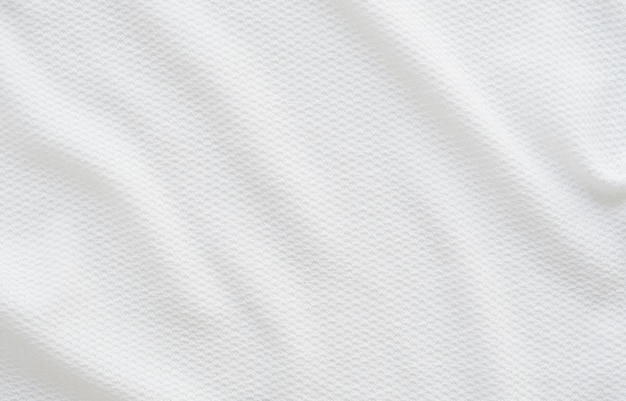This close-up photograph captures a section of white fabric with a distinctive waffle weave, characterized by its octagonal mesh design. The texture reveals a slightly bumpy, thicker cotton material, possibly part of a waffle hooded drawstring hoodie. The fabric surface exhibits multiple wrinkles, creating varying heights and shadows, adding depth to the image. Notably, there are prominent wrinkles in the upper right-hand corner and several extending from top to bottom, and on the left side. The intricate mesh pattern covers the entire frame, making the material appear as though it has small hills or mountains, and the weave itself resembles a honeycomb, contrasting with the otherwise smooth texture.